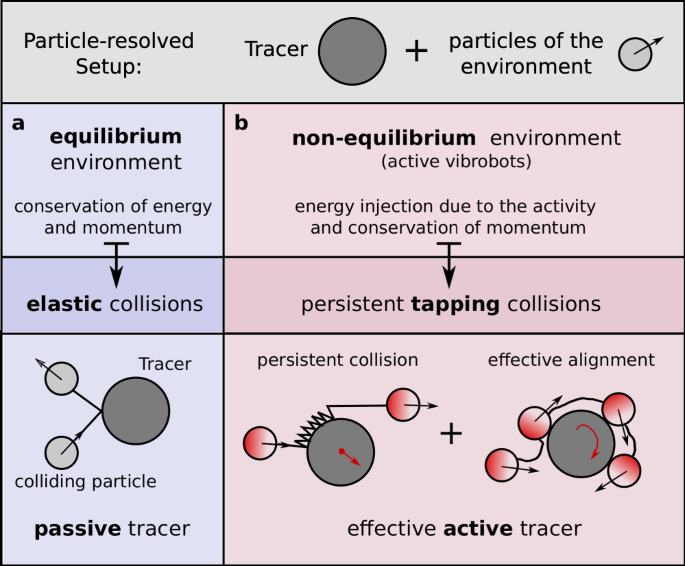The image displayed is a detailed, scientific chart likely from a textbook or conference poster, titled "Particle Resolved Setup". The chart is divided into two columns, A on the left and B on the right. At the top, it features a gray circle labeled "Tracer" alongside a plus sign next to "Particles of the Environment," denoted by a smaller gray circle.

Column A represents the "Equilibrium Environmental Conservation of Energy and Momentum," with an arrow pointing down to "Elastic Collisions" and a series of circles depicting a large central circle with arrows radiating outward to smaller circles. This setup illustrates the concept of a "Passive Tracer," where the tracer collides within the environment maintaining equilibrium.

To the right, Column B details the "Non-Equilibrium Persistent Trapping" environment, characterized by "Effective Active Tracer." It mentions "Persistent Collision plus Effective Alignment," indicating processes influenced by persistent interactions and alignment of particles.

Overall, the chart serves as a comparative illustration of equilibrium versus non-equilibrium environments and their impact on particle behavior, notably between passive and active tracers.